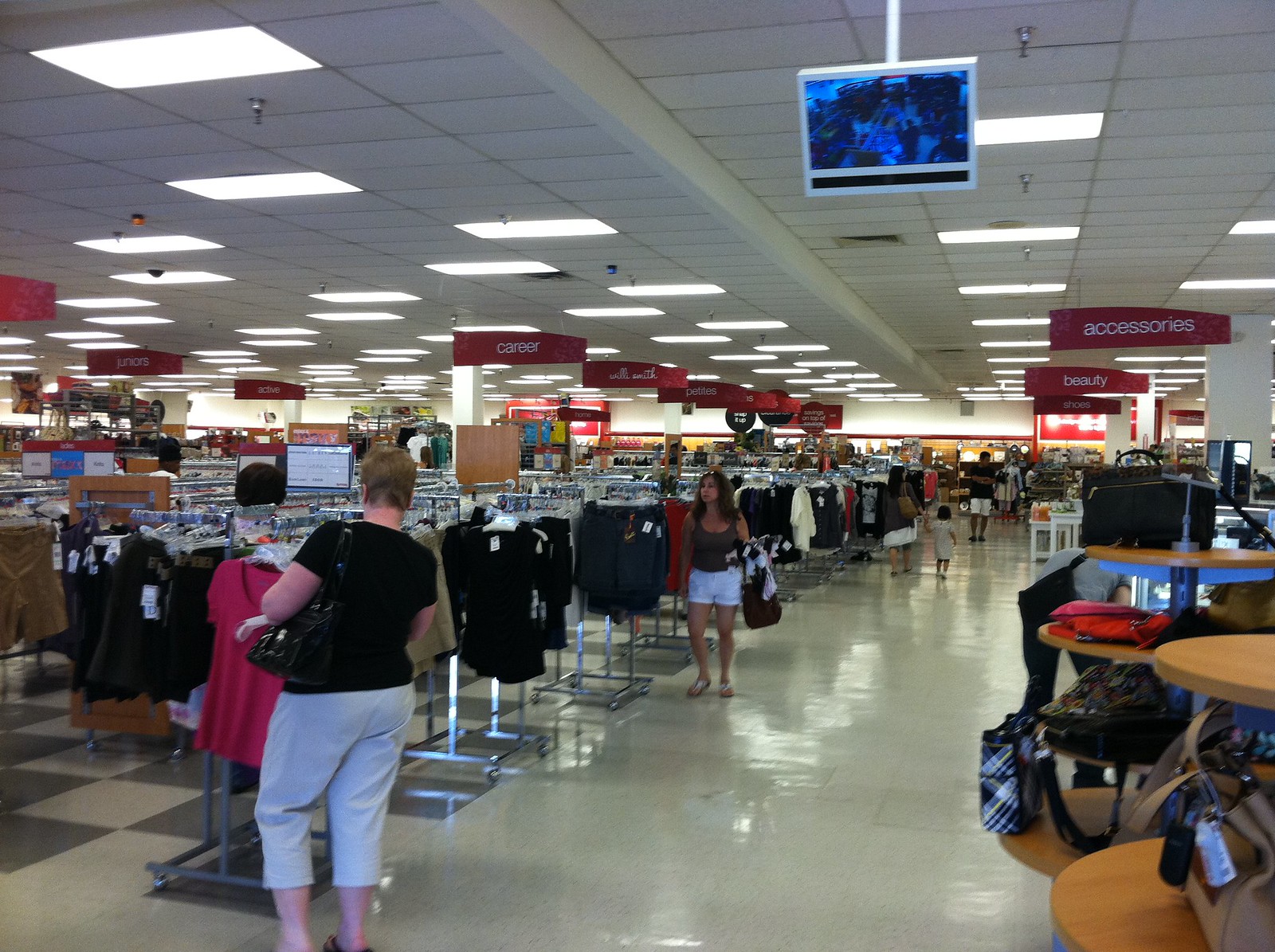This detailed color photograph captures the interior of a department store, specifically within the women's clothing section. The store features a shiny, cream-colored floor with gray squares and a white ceiling composed of foam tiles, interspersed with clear plastic ones that house light sources. The ceiling also has small silver sprinkler heads. Red signs with white lettering hang from the ceiling, indicating different departments such as career, petite, beauty accessories, and other categories, enhancing the navigability for shoppers.

The aisle is busy with several people; some are walking while others are standing and examining the various items. Clothes racks are filled with an assortment of garments in colors such as red, blue, black, and tan, each adorned with white tags. On the right side, brown wooden display racks hold an array of purses, organized in a tiered, circular fashion, with sizes decreasing from bottom to top. The purses come in shades of red, tan, black, and blue. A white security monitor suspended on a pole from the ceiling displays a live feed of the store floor on a blue screen, contributing to the store's security measures.